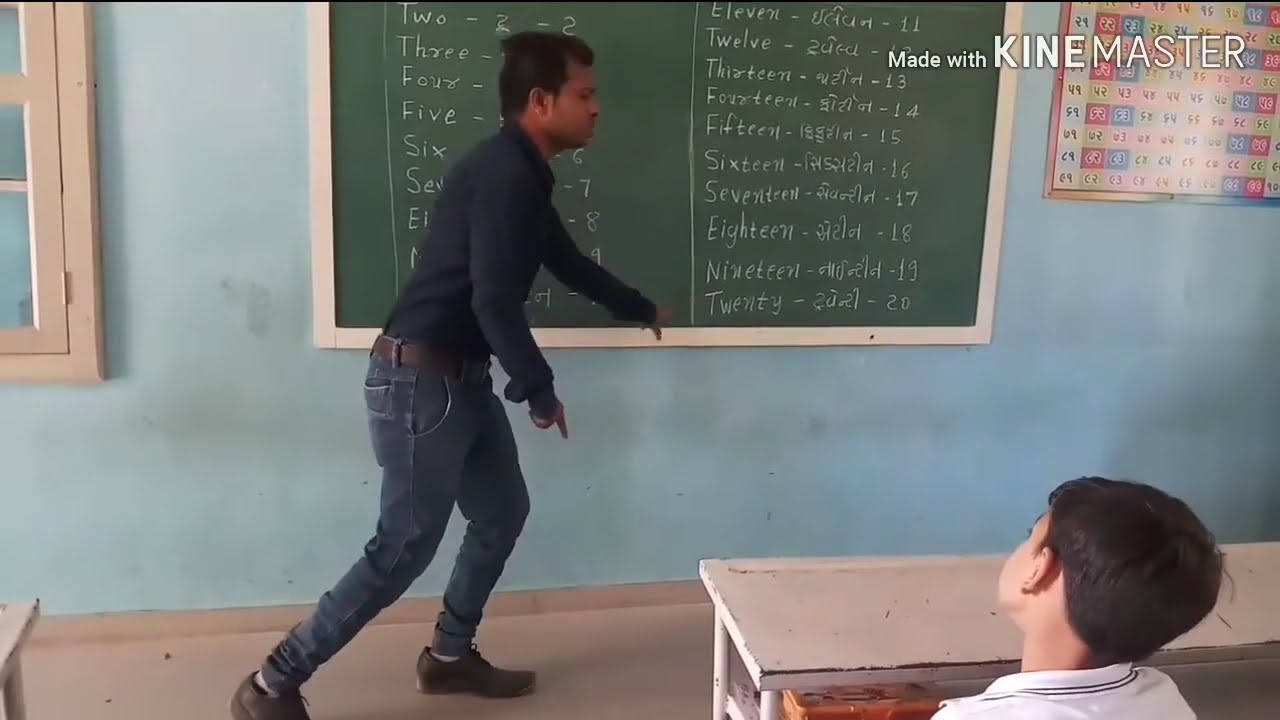The image captures a dynamic moment in a classroom setting, appearing to be a screen grab from a video made with KineMaster, as indicated by the text in the upper right corner. The focal point is a young man, presumably a teacher in his early 20s, of South Asian descent, with a darker complexion and short black hair. He is dressed in a long-sleeve navy blue shirt, dark blue jeans secured with a brown belt, and brown shoes. He is in front of a green chalkboard covered with numbers written in both English and another language, possibly Arabic or Indonesian, and numerical symbols ranging from 2 to 20. 

The teacher is caught mid-action, walking to his right with an unusual posture, one hand potentially interacting with the chalkboard while the other points. The classroom features light blue walls and a wooden floor. A white desk positioned in the bottom right of the image supports a young boy in a white shirt with short dark brown hair, who is intently watching the teacher, his head slightly tilted to the right. Additionally, a poster listing numbers up to 100 in small font is visible at the top left, adding to the educational atmosphere of the room.